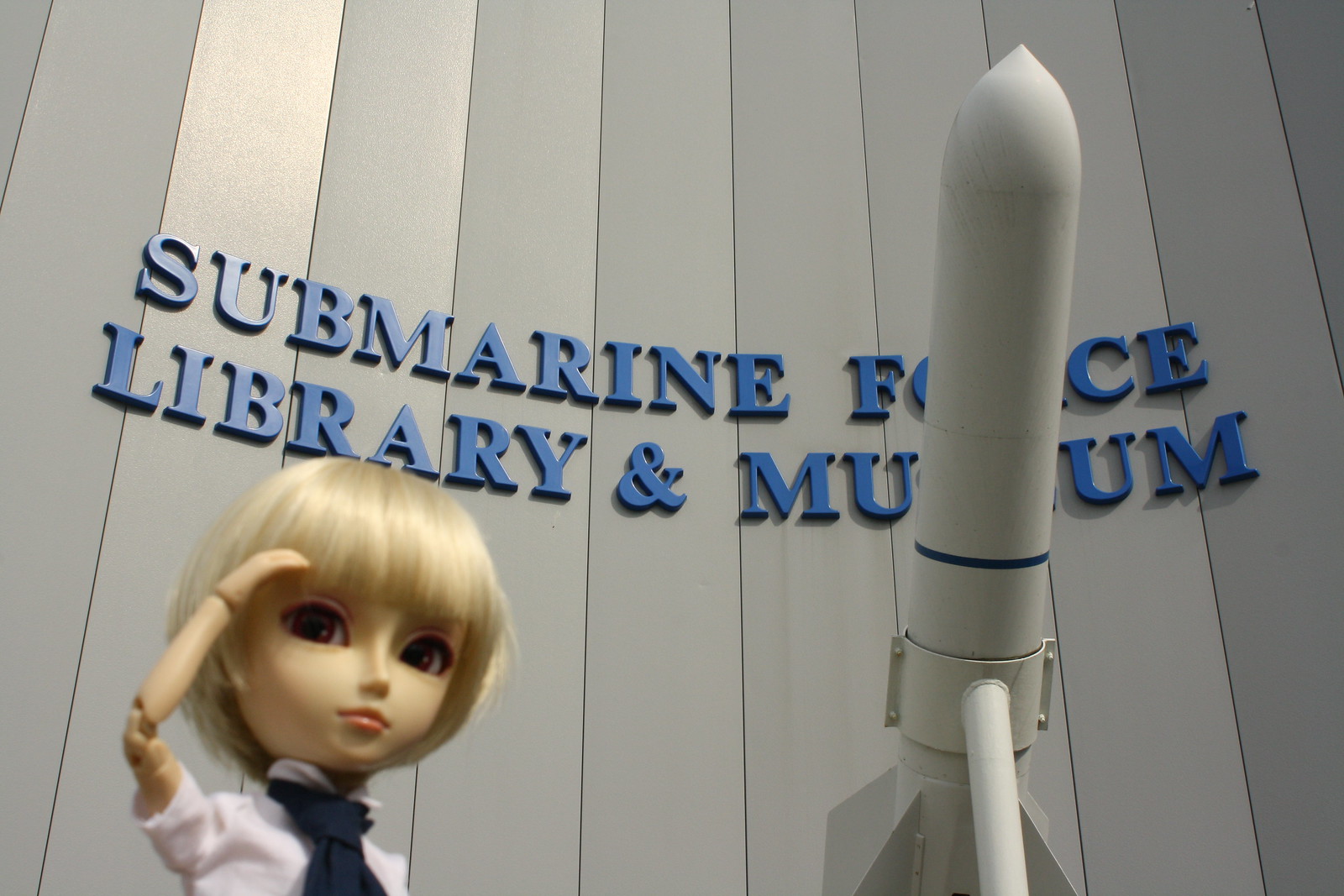The image captures an exhibit at the Submarine Force Library and Museum. Central to the foreground on the left is a doll reminiscent of a Team America or Bratz figure, characterized by prominent features such as large eyes, a small nose, and a large head relative to its body. The doll, standing and saluting with its right hand, is dressed in a white short-sleeved button-down shirt paired with a large blue tie, and has short blonde hair styled in a bowl cut. Adjacent to the doll on the right, there is a gray warhead missile positioned pointing upwards, secured on a stand. The backdrop of the exhibit features a gray wall with vertical slat panels, embossed with the blue capital-lettered inscription "SUBMARINE FORCE LIBRARY AND MUSEUM."